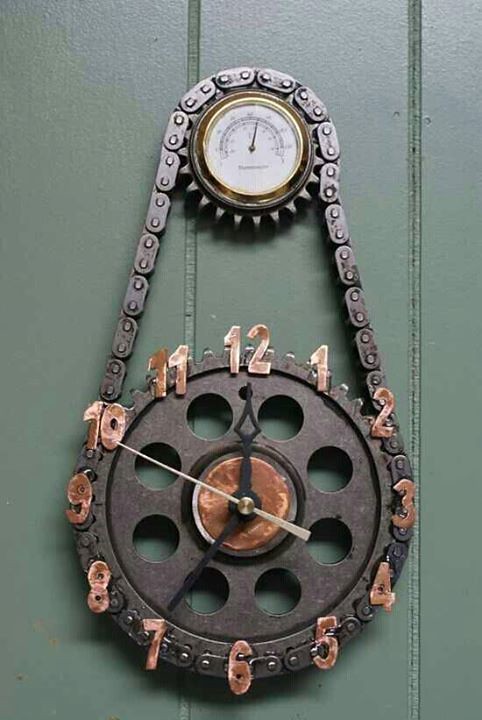This image showcases an artistic wall clock with a captivating industrial design aesthetic, set against a green painted wooden background composed of vertically placed boards. The clock, which seems to be constructed from mechanical parts and machinery components, incorporates a large gear as its main body, with the numbers 1 through 12 attached unevenly around its perimeter, contributing to its rustic and handcrafted charm. These numbers, potentially made of copper or a similarly colored metal, exhibit patterns enhancing the piece's vintage feel. Centrally, a smaller gear or circular plate, featuring a coppery disc, serves as the backdrop for the classic-style clock hands, positioned at 10 minutes past 10 o'clock. Above the clock, a barometer with an analog needle and a white background, encircled by a gold-painted border, adds a functional yet ornate touch. Additionally, a bicycle chain creatively connects the barometer to the clock below, further emphasizing the industrial and recycled art theme, with the clock's design hinting at a bicycle spoke structure.